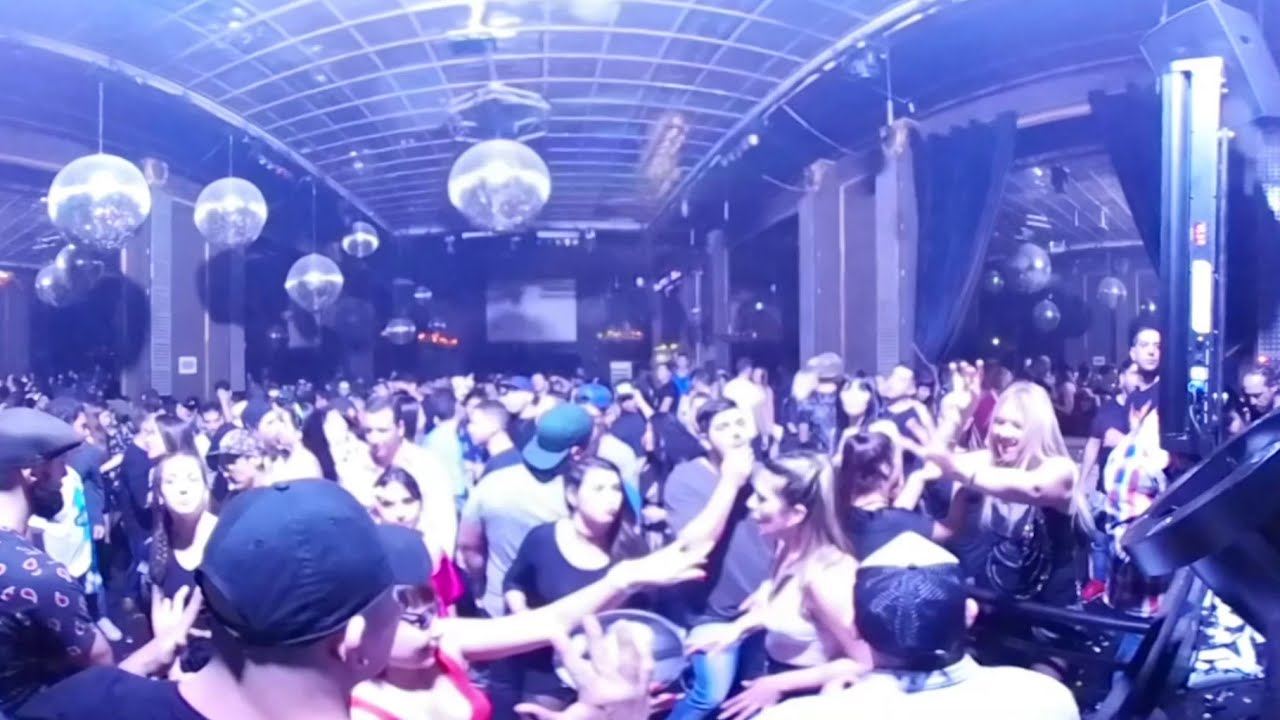The image captures a vibrant and crowded club or disco event in a large ballroom-style room with a glass-like or reflective ceiling. The top of the ceiling is adorned with numerous disco balls — at least six to eight — hanging down primarily on the left side but also visible in other areas of the room. The right side of the image features curtains that seem to open up to another area or room, also adorned with similar disco balls. The focal point of the image is the densely packed crowd, with people standing so closely that there is very little room between them. Many of the attendees are wearing baseball caps or hats, predominantly in colors like black or dark blue.

In the bottom left, partially obstructed by the crowd, are two individuals: one, a person with a ball cap seen from the neck up, and another beside them visible from the shoulders up, both looking away from the camera. Above them, slightly to the right, a woman is facing the camera with her arm extended outward. The crowd is animated, with people waving, pointing, and socializing, giving the impression that they are enjoying themselves. The back of the room features a large screen displaying dance music visuals, set against a black wall, with the ceiling decorated with club-style lighting and possibly stage setups. Overall, the image conveys a lively atmosphere filled with dancing, mingling, and a nearly equal ratio of males to females, all immersed in the high-energy ambiance of the event.